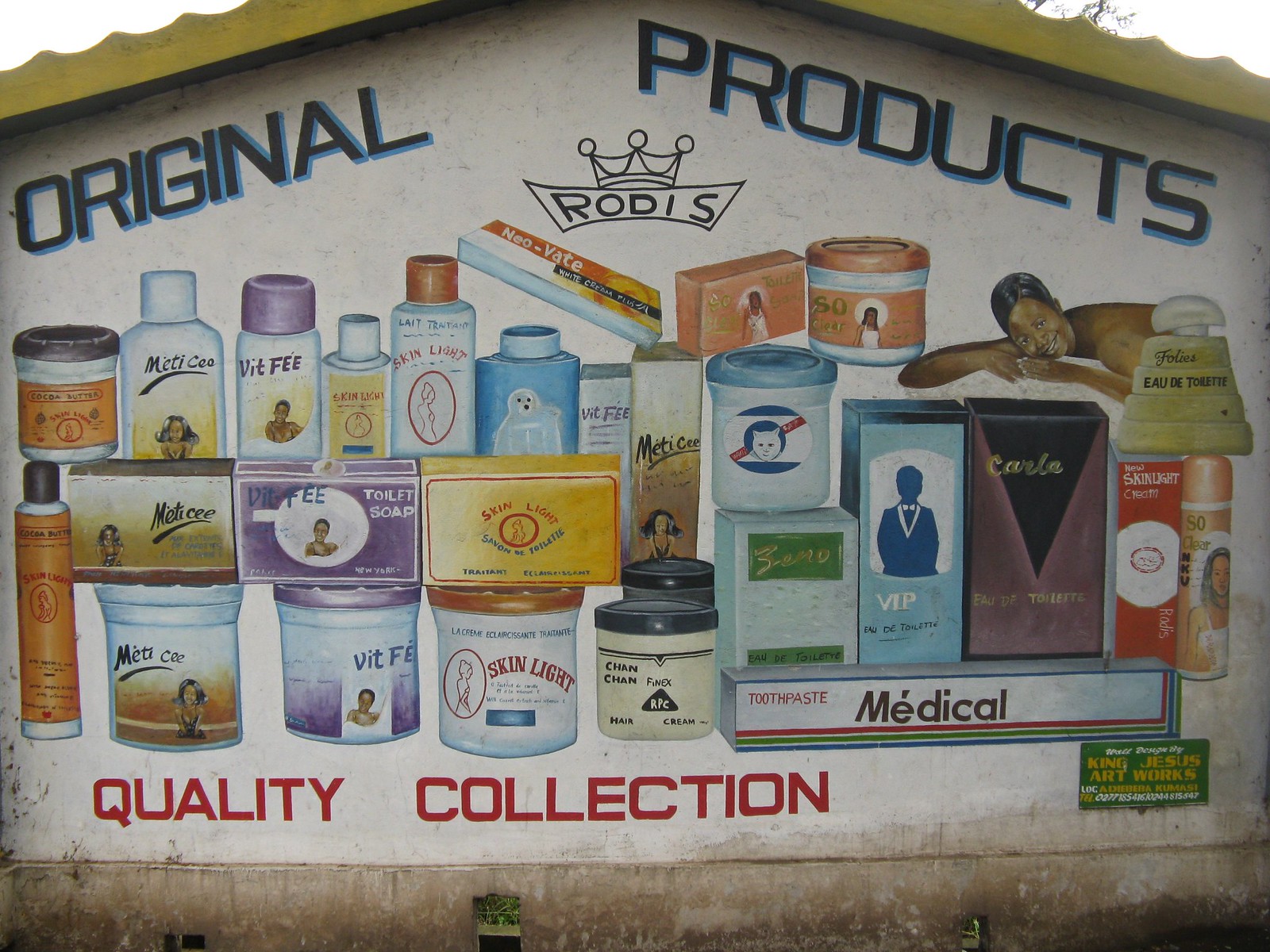This image depicts an old-style advertisement painted on the side of a white building with a yellow roof barely visible. Dominating the side of the structure is a colorful mural showcasing a collection of beauty and self-care products. At the top of the mural, in blue text, "Original Products" is prominently displayed. Centered below this header is a black logo featuring a crown and the brand name "Rodis." The mural includes a variety of painted product illustrations, including items labeled "Metixi," "Ditfi," "Skinlight," and "Chan Chan," featuring toilet soap, skin lightening products, and toothpaste. An additional product, "Eau de Toilette," is also visible. At the bottom of the advertisement, in red font, it reads "Quality Collection." The mural suggests these products may be of foreign origin, possibly older and unfamiliar in North America. In the bottom right corner of the mural, the text "King Jesus Artworks" indicates the artist behind this vibrant, nostalgic display.